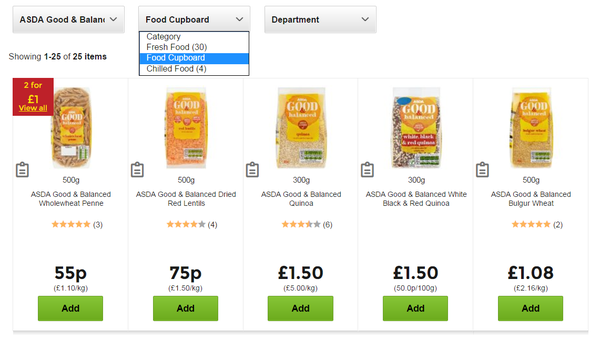The image features a webpage with a white background and several organized drop-down boxes. At the top, two prominent gray drop-down boxes are displayed: one reads "ASDA Good and Balanced," and the other reads "Food Cupboard." Below these, a gray box labeled "Department" is visible, accompanied by a category drop-down suggesting options such as "Fresh Food 30," "Food Cupboard," and "Chill Food 4."

Below these boxes are listings of five different products from the ASDA Good and Balanced line, described in detail from left to right:

1. A package of whole wheat penne, weighing 500 grams, priced at 55 pence (1.10 per kilogram). It boasts a rating of 4.3 stars based on 5 reviews and includes a promotional offer: "2 for 1 pound." A green button marked "Add" is available for purchasing the item.
   
2. A package of dried red lentils, also weighing 500 grams, priced at 75 pence (1.50 per kilogram). This product has received a 4-star rating based on 4 reviews. A green "Add" button is shown adjacent for adding the item to the cart.

3. A 300-gram package of quinoa, priced at 1 pound and 50 pence (5 pounds per kilogram). It has a 3.5-star rating from 6 reviews and features a green "Add" button for easy purchase.

The detailed descriptions and clear layout make it convenient for users to select and add products to their carts based on their ratings, quantity, and price per kilogram.